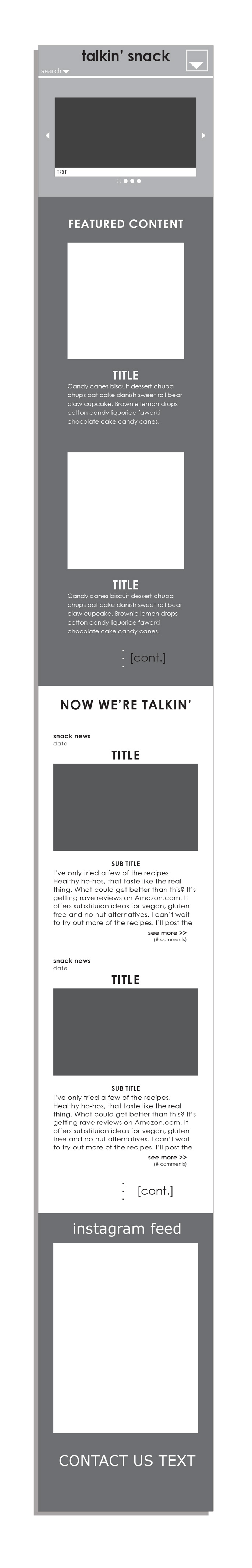This image is a screenshot of a prototype for a website, displaying a simplistic and content-light layout. The design is segmented into four distinct sections, each shaded differently to demarcate their functions. 

1. **Header Section (Light Gray)**: This portion likely serves as the header, possibly featuring space for a video or introductory content.
2. **Featured Content Section (Dark Gray)**: This segment is labeled "Featured Content" and includes a couple of title cards accompanied by descriptive text below each card.
3. **Additional Content Section (White)**: This area also contains headers and title cards, with allocated spots for images and accompanying text to provide further information.
4. **Footer Section (Dark Gray)**: The footer houses an Instagram feed, a placeholder for an image or logo, followed by a "Contact Us" prompt for user interaction.

The varying shades of gray and white backgrounds help to visually separate and organize the website's content.